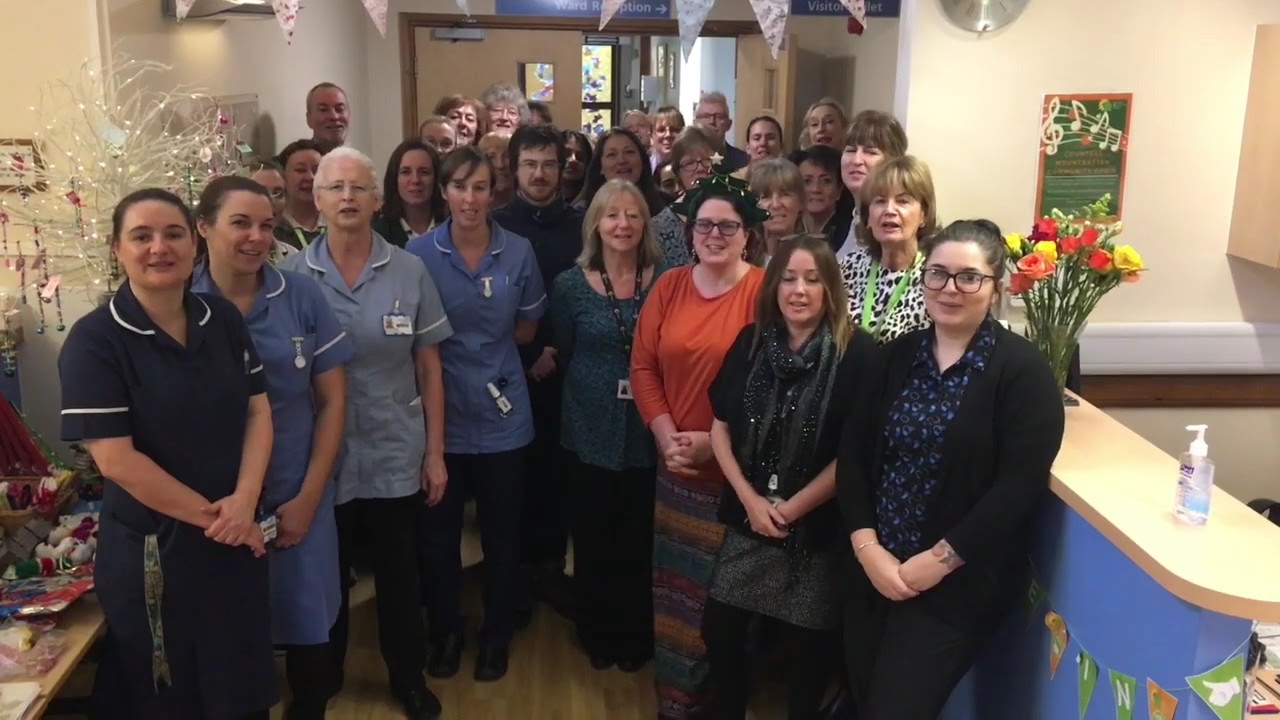The photograph captures a group of over 20 individuals who appear to be staff at a healthcare facility, potentially a hospital, nursing home, or doctor's office. The majority of the people in the image are women, although there are some men standing behind them. Many of the individuals are wearing National Health Service (NHS) uniforms in varying shades of blue, which consist of short-sleeved, long button-down shirts or dresses with white piping and dark blue trousers. The crowd is standing in front of a reception counter adorned with a vase of bright flowers in red, yellow, and orange. Decorative elements, including a small Christmas tree with white lights and branches, as well as a surface with packaged pastries, are visible to the left. There is a banner hanging from the ceiling, partially obscured, indicating some form of celebration or event. In the background, a set of double doors leads to another room, emphasizing the busy yet festive atmosphere of the facility.